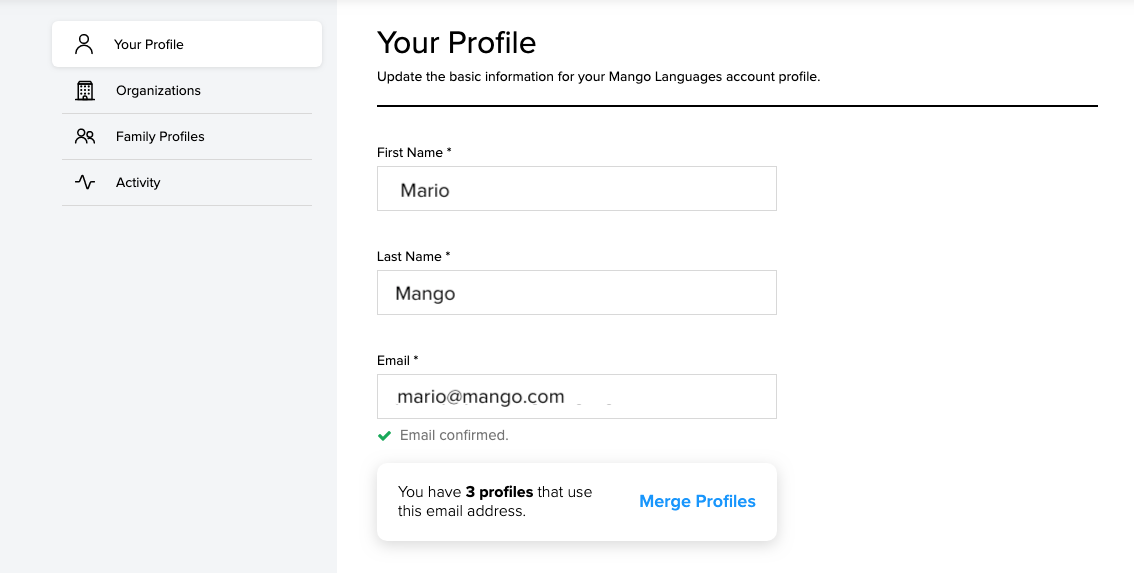Screenshot of Mango Languages User Profile Management Interface

The desktop screenshot depicts the user profile management interface of the Mango Languages platform. On the left-hand side, there is a light gray vertical sidebar with various navigation options. 

- The highlighted selection is "Your Profile," represented by an androgynous pictogram of a figure.
- Below it, an icon of a building accompanies the "Organizations" option.
- "Family Profiles" is the next option, illustrated with a similar figure pictogram, depicting a smaller figure alongside a larger one.
- Lastly, the "Activity" section is indicated by an icon that resembles either a sideways 'Z' or a heart rhythm monitor.

In the central area of the screenshot, the interface displays detailed information under "Your Profile," where users can update their basic details. Here, the first name "Marco" and last name "Mango" are shown, along with the email address "mario@mango.com," which has been confirmed. Given the coincidental surname of the profile holder, it is likely a demo account.

At the bottom, it is noted that there are "three profiles that use this email address," with an actionable blue button labeled "Merge Profiles" available to the right.

This detailed view makes it clear that the interface is part of a user account management system, specifically for Mango Languages.